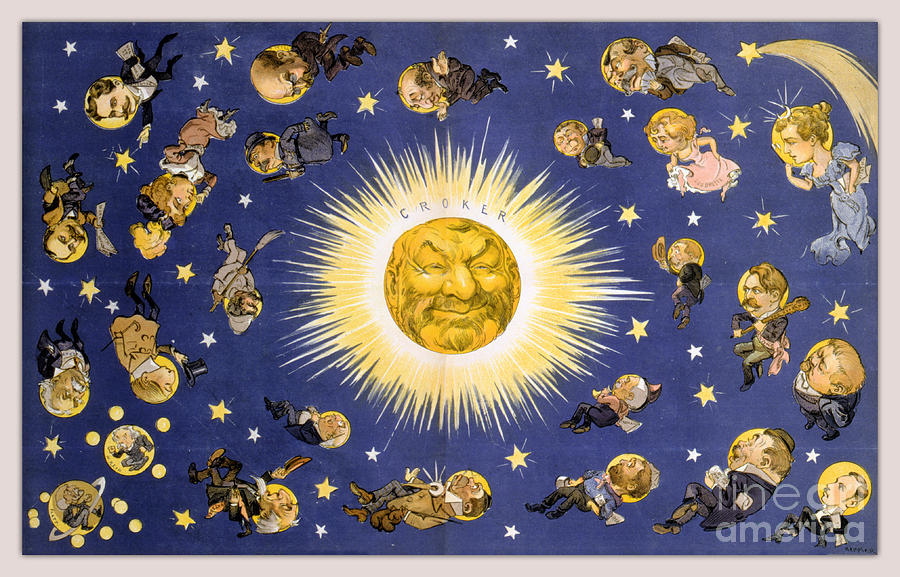This color illustration, drawn in an old comic-style, features a central Sun with a slightly smiling aged man's face, detailed with a large nose, goatee, and mustache. Above the Sun, in black letters, is the word "CROKER." The Sun radiates yellow and white light into a dark blue background sprinkled with yellow and white stars, including a yellow shooting star in the upper right corner leaving a trail. The entire scene is bordered by a thin white frame. Surrounding the Sun, in a circular pattern, are multiple rows of floating, cartoonish illustrations of famous historical figures and other characters, dressed in old-fashioned clothing. Among the floating people, one can recognize notable faces such as Albert Einstein in the bottom left, a character resembling Sherlock Holmes, and a figure that looks like Franklin D. Roosevelt. Men predominantly wear pants and suit coats, often sporting old-fashioned mustaches, while women are depicted in various dresses, including a blue and a pink one. The overall whimsical appearance of the artwork captures a celestial and historical convergence with a playful, vintage flair.